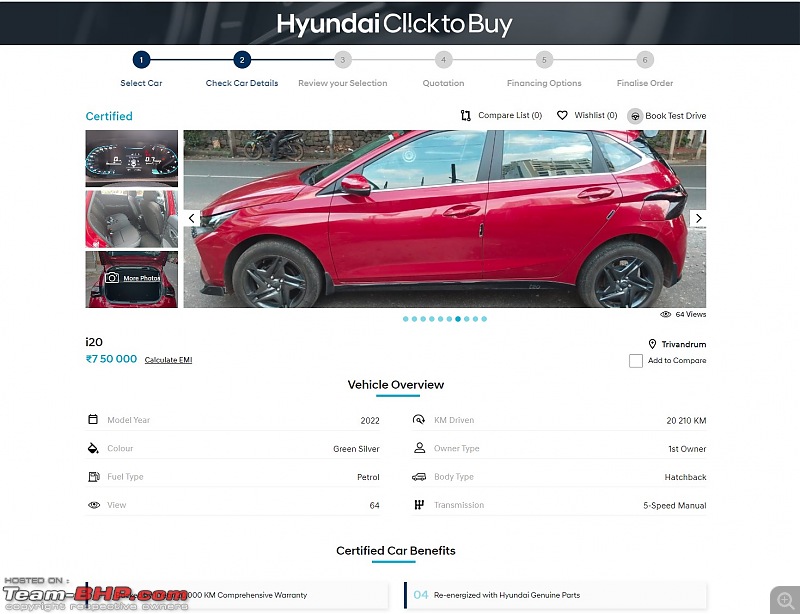The image is a snapshot of an online car buying webpage from the website team-bhp.com. At the top, the text "Hyundai, Click to Buy" is prominently displayed in white font. Below the text is a profile view of a small red hatchback car with four doors and black rims. The photo provides a glimpse of the car's interior, showing part of the back seat, as well as a small view of the open trunk and the vehicle's dashboard, including the speedometer.

Further down the page, the vehicle overview section provides detailed information about the car. It lists the model year, color, fuel type, body type, owner history (indicating that it has had only one previous owner), and the transmission type, which is a 5-speed manual. The number of views the car has received from potential buyers is also displayed. Overall, the webpage offers comprehensive details and visuals to assist users in purchasing a car online.